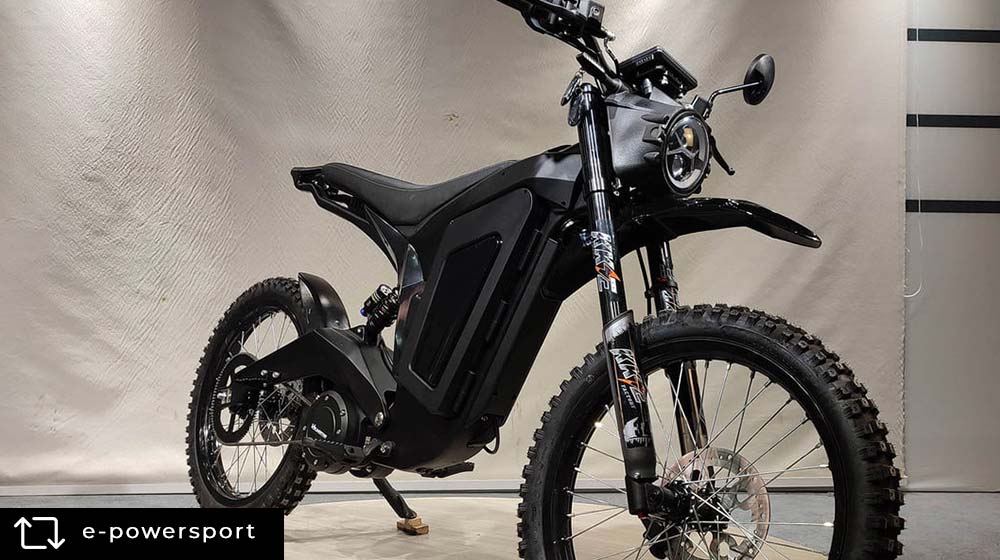In this detailed color photograph with a landscape orientation, a sleek black motorbike is the central subject. The motorbike, with its angular, flat black body panels and minimal curves, exudes a modern and edgy aesthetic. Its knobby, fat-walled tires suggest it’s built for rugged use. The motorbike leans slightly to the right, stabilized by its kickstand. The front tire is oriented toward the bottom right corner, while the rear tire points to the left. 

The front of the bike features silver accents, including a chrome-covered headlight and rearview mirrors. A notable detail is the elevated black fender above the front tire. The motorbike rests on a surface that blends light gray flooring with a beige mat or tarp directly beneath it. 

In the background, part of the wall is adorned with a white fabric, adding texture to the scene. The upper right section of the wall displays horizontal black stripes, contributing to the photograph's stark contrast. On the bottom left corner of the image, a black banner with a white logo—a box formed by two arrows pointing up and down—and the text "e-Powersport" in lowercase letters is prominently displayed. The style of this image aligns with photographic realism, capturing the motorbike and its surroundings with clear, precise detail.